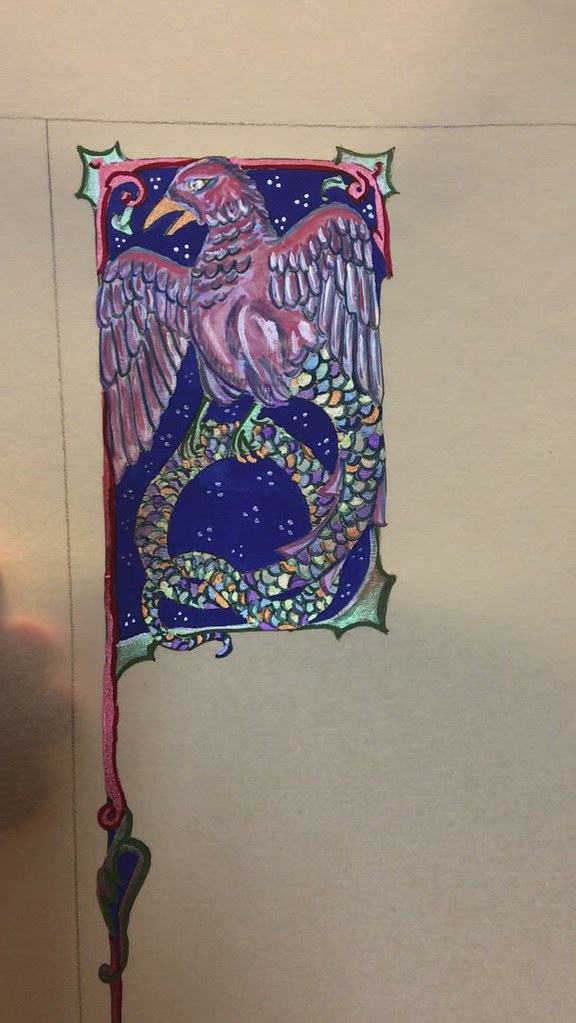This vibrant drawing showcases a meticulously detailed, small-scale depiction of a bird. The bird, predominantly reddish in color with an orange beak, is skillfully illustrated within a square frame. Its wings are spread wide, revealing an array of white feathers interspersed with dazzling hues. Most striking is the bird's extraordinarily long, snake-like tail, which it appears to grasp with its talons. This tail, vividly adorned with blue, green, purple, and orange scales, intricately entwines upon itself, lending a serpentine charm to the piece. The overall composition, brimming with diverse colors and fine details, transforms a simple doodle into a captivating work of art.